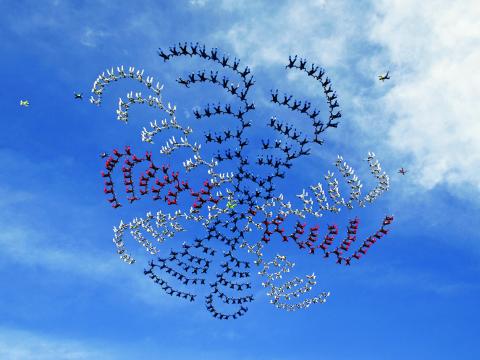The photo captures a striking aerial spectacle set against a medium blue daytime sky with distant white clouds. The focal point is a group of skydivers who have formed a synchronized, spiral floral pattern by holding hands, reminiscent of artistic expressions such as synchronized swimming. The participants are wearing uniforms in varied colors—white to silver, dark blue, and magenta—contributing to an abstract visual effect. The formation is slightly out of focus, adding to the dreamlike quality of the scene. Additionally, small planes can be discerned entering from both the right and left sides of the image, suggesting they are coordinating or observing the skydivers’ performance. The overall effect is one of harmony and precision, as the skydivers in black, white, and red uniforms create a dynamic and mesmerizing X-shaped floral design against the serene backdrop.